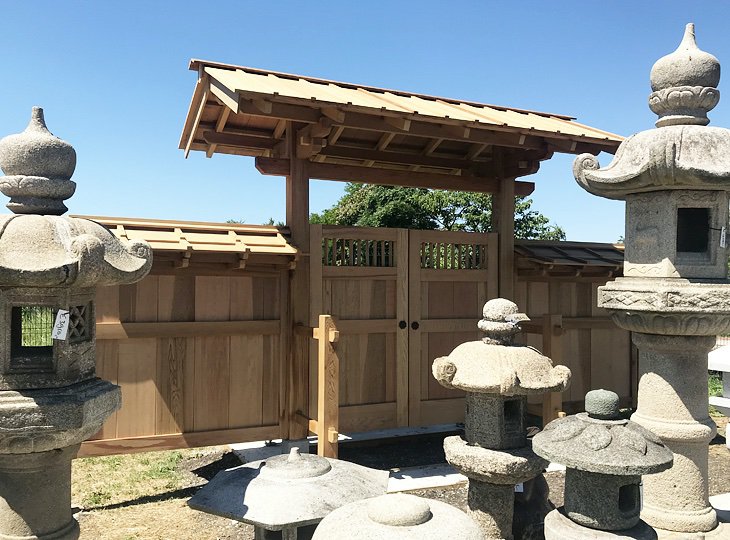This photograph captures a collection of Japanese-style garden ornaments made of concrete, arranged in what appears to be an outdoor display area. The scene is set on a sunny day, with a clear blue sky that illuminates the garden items. These concrete structures, which resemble primitive pagodas or lanterns, showcase a blend of simplicity and elegance without intricate designs. There are two taller structures and four shorter ones, all distinct in their appearance and standing side by side on what looks like a dirt lot. Price tags on a couple of the items suggest they are for sale. In the background, there is an impressive wooden fence with a swinging gate, characterized by traditional Japanese architectural elements, including a distinctive triangular roofing structure. The setting evokes a serene, garden-like atmosphere, enhanced by the presence of a tree outside the enclosure and the clear sky above.